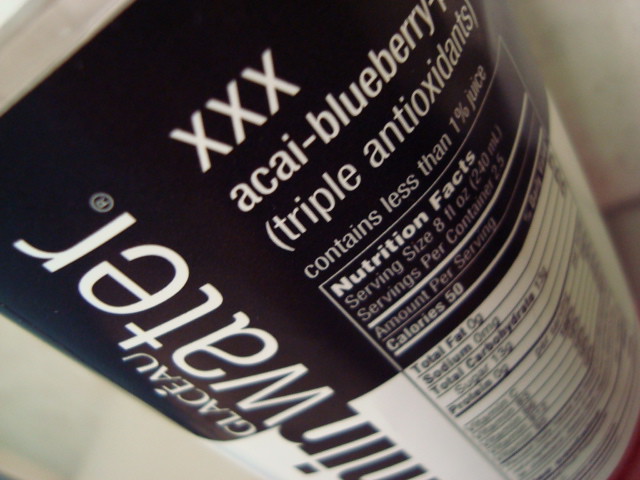The image features a plastic bottle of Vitamin Water, prominently labeled with "Vitamin Water" in bold white and black text on a white background. The label also displays the flavor, "Aku Blueberry," and highlights its claim of being "Triple Antioxidant" in white text against a contrasting background. The bottle appears half full, containing a deep red liquid. Nutritional information, including details on fat, carbohydrates, and other nutritional facts, is clearly printed in black lettering on the white label. The perspective of the image is a top-down view, emphasizing the branding and the partially filled state of the bottle.